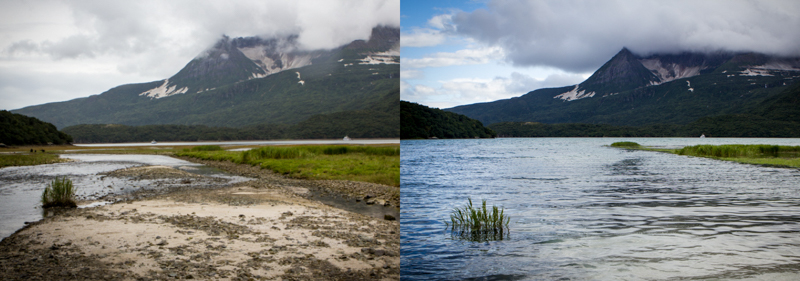This rectangular image is a side-by-side comparison of two photographs of the same location taken at different times. Each photograph occupies 50% of the overall image. Both show a landscape dominated by the impressive Skame Mountain in the distance, which is covered with dark green vegetation and has patches of light gray rock. 

The photograph on the left features a body of water that has mostly dried up, exposing large clumps of land and sand. The mountain appears under a cloudy and gray sky, creating a dull and desaturated look. In contrast, the photograph on the right shows a revitalized scene where the body of water is filled up, covering much of the previously visible sand. The sky is blue with scattered white clouds, adding vibrancy to the image. The consistent elements between the two photographs include the mountain, its vegetative cover, and the body of water, making the changes in weather and water levels starkly noticeable.